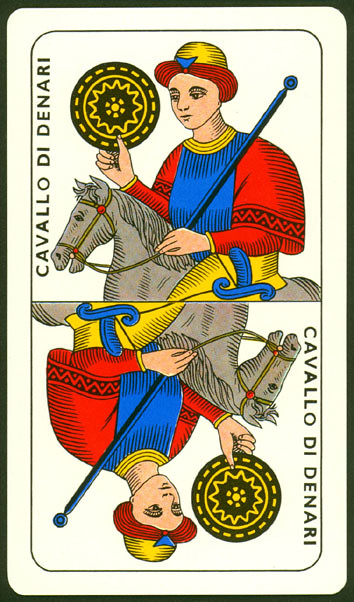This image features a detailed representation of a playing card set against a black backdrop. The card itself has rounded edges and is predominantly white, emblazoned with the name "Calo de Denari." The card is illustrated with a vibrant design of a man astride a gray horse, dressed in a colorful outfit comprising yellow, blue, and red garments. The man holds a blue staff in his left hand and a black shield adorned with a yellow pattern in his right. He wears a distinctive hat that has a yellow crown, a red brim, and a blue central piece on the forehead. The card is mirrored such that if flipped, the image and the text "Calo de Denari" would align with the opposite side, forming a continuous depiction of the character and his regalia.